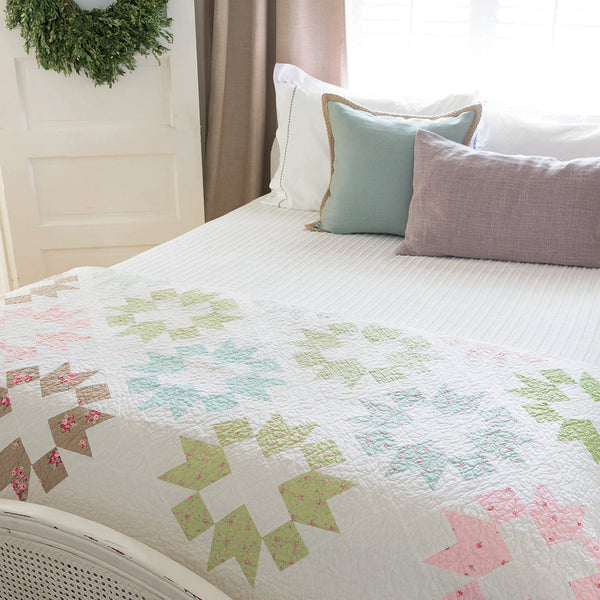This image depicts a well-made bed in a cozy bedroom, captured from the footboard towards the headboard. The bedspread is predominantly white with a textured striped design, complemented by a folded blanket at the foot featuring intricate plus sign and snowflake-like patterns in light blue, light green, pink, and brown. The bed is adorned with multiple pillows: two white ones at the back, a square aqua-colored one, and a longer pillow in a shade of salmon or light purple.

The white bed frame at the foot of the bed is distinctively arched with a pattern of small holes, giving it a decorative, vent-like appearance. To the left of the bed is an open white door with a green wreath hanging on it. Behind the bed, natural light streams in through a window, filtered by brownish or light brown curtains. The bright atmosphere is completed by the overall neatness of the room, suggesting it might be a staged setup for an advertisement or simply a snapshot of a tidy, inviting bedroom.